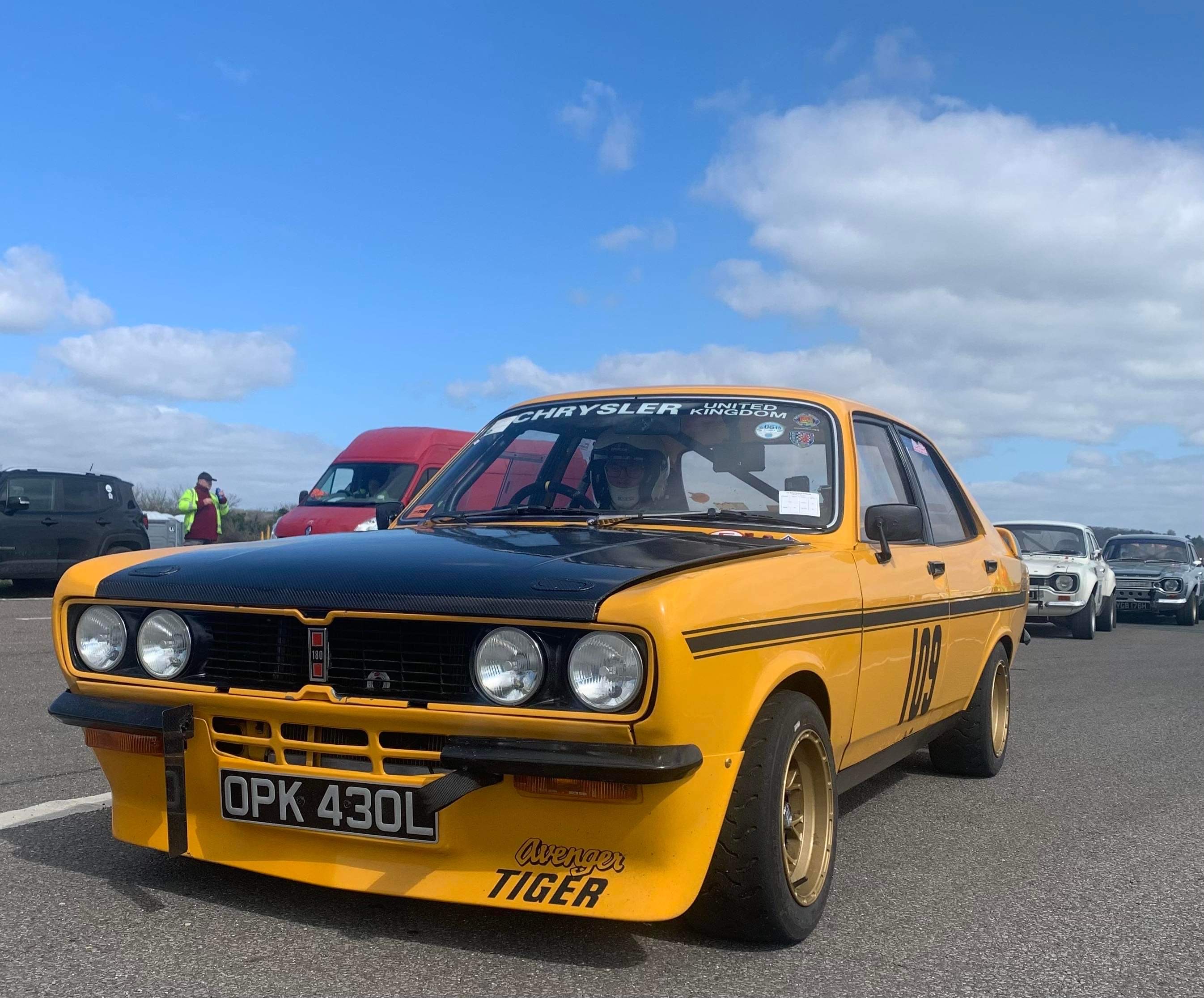In this vibrant photograph, the centerpiece is a vintage yellow race car prominently displaying the name "Avenger Tiger" on its left front bumper. The car, adorned with a bold black stripe flanked by two thinner black stripes running along its sides, carries the number 109 in black on its driver's door and hood. The front of the car reveals a license plate reading "OPK430L" on a black background with white uppercase letters. At the very top of the front window, "Chrysler United Kingdom" is inscribed in white. The hood of the car is strikingly black, adding contrast to its predominantly yellow body. Situated behind the yellow car, four other vehicles—one dark blue, one white, one dark red, and one black—are partially visible, fading into the background. An individual in a white helmet is in the driver's seat of the yellow car, ready to race. Additionally, a man in a yellow jacket stands near a black SUV to the left, while the blue sky overhead is dotted with a few white clouds, setting a picturesque backdrop for this dynamic scene.